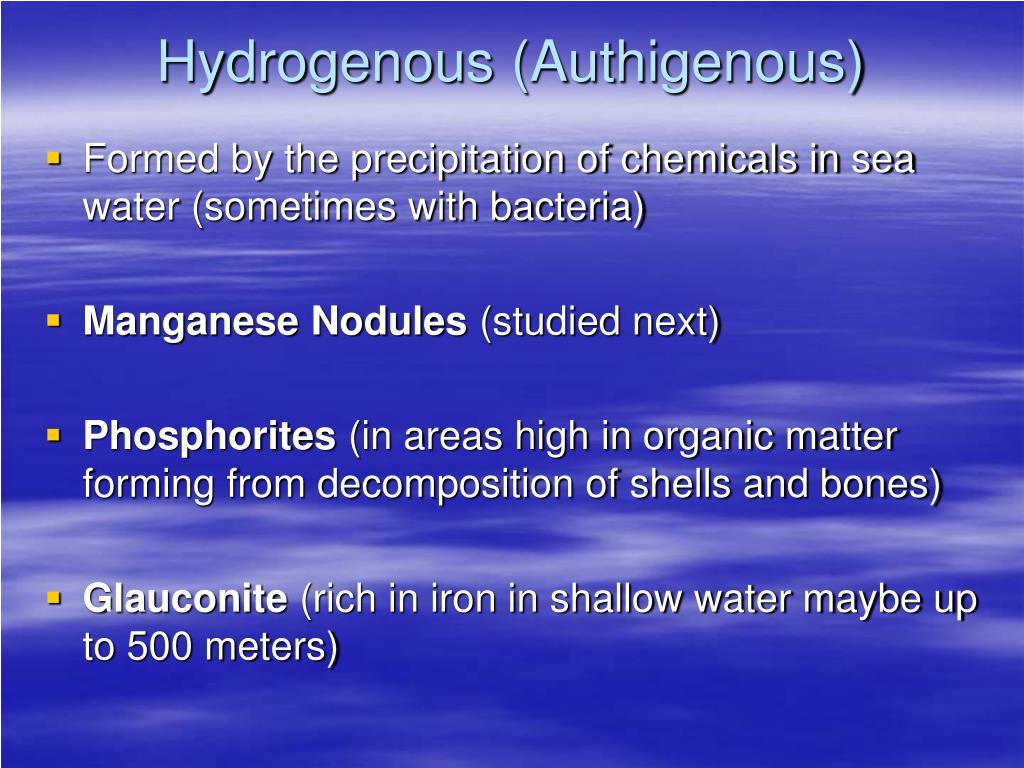The image is an infographic designed to resemble a sky with thin, white clouds set against a blue background, suggesting a sky view from an airplane window. At the top center, light blue text reads "Hydrogenous" and "Altegenous" (or "Othogenous"). Below, there are four bullet points written in white text, each marked with gold-colored square bullets. The points read: "Formed by the precipitation of chemicals in seawater, sometimes with bacteria," "Manganese nodules, studied next," "Phosphorites, in areas high in organic matter forming from decomposition of shells and bones," and "Glauconite, rich in iron, in shallow water, maybe up to 500 meters." This infographic appears to be a PowerPoint presentation slide focused on geological formations.